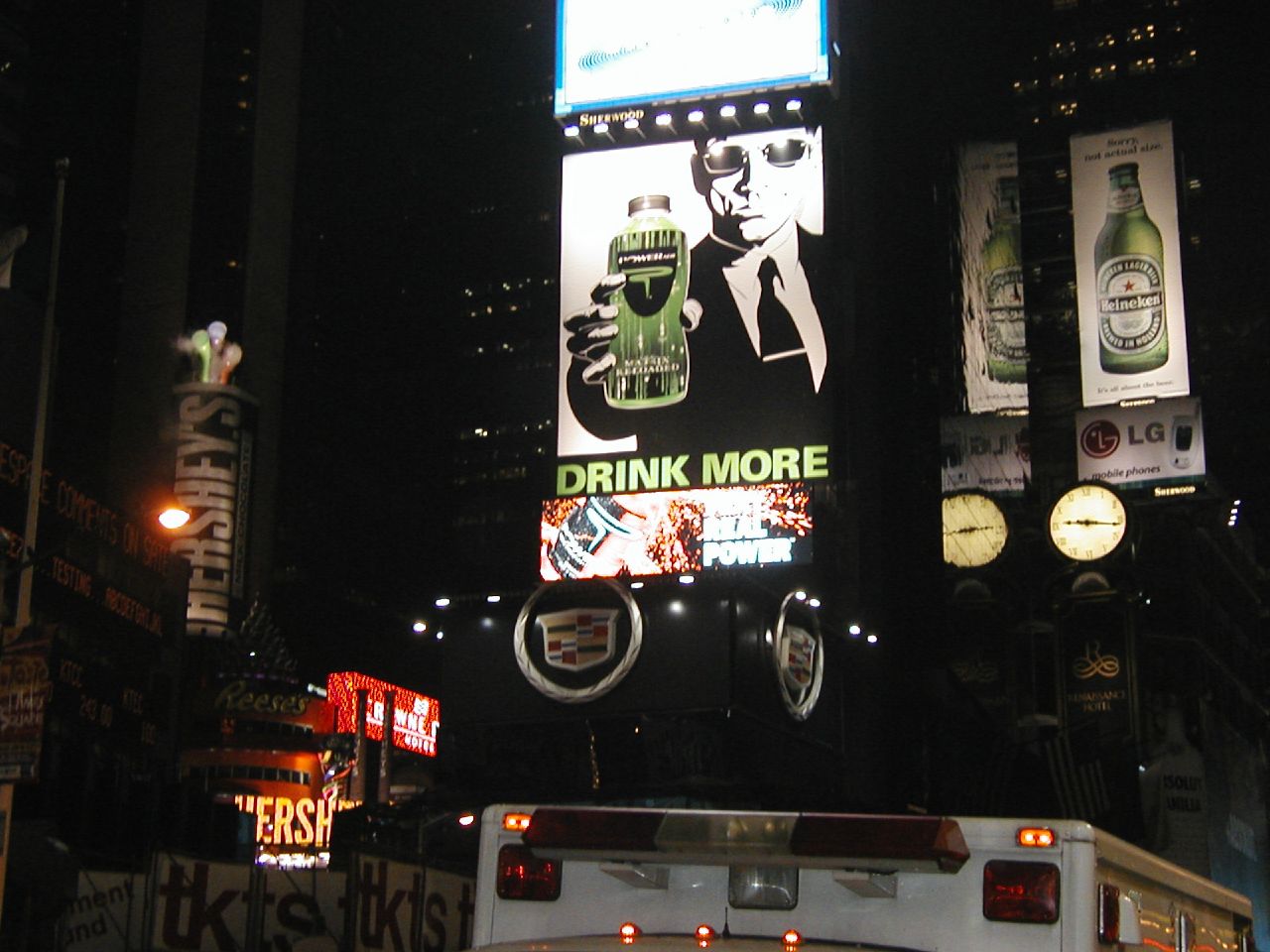This is a nighttime cityscape photo, likely in New York City, featuring a bustling array of billboards and advertisements. At the very bottom of the image, the top of an ambulance, distinguishable by its lights, is visible. Dominating the scene are various advertisements: centrally, there's a prominent black and white ad featuring a man in a suit and tie with sunglasses, holding out a Powerade drink, accompanied by the slogan "Drink More." To the right, there's a Heineken beer bottle ad. Below the Heineken billboard is an LG advertisement, and beneath it, a grandfather clock with a round face. To the left of the Powerade ad, there's a large Hershey's bar billboard, accented by Reese's and some balloons. Underneath the Hershey’s ad is a sign for TKTS, which stands for tickets. A Cadillac symbol atop the clock, a Buick logo, and the lit-up office windows in the distant skyscrapers add to the vibrant atmosphere of the scene.